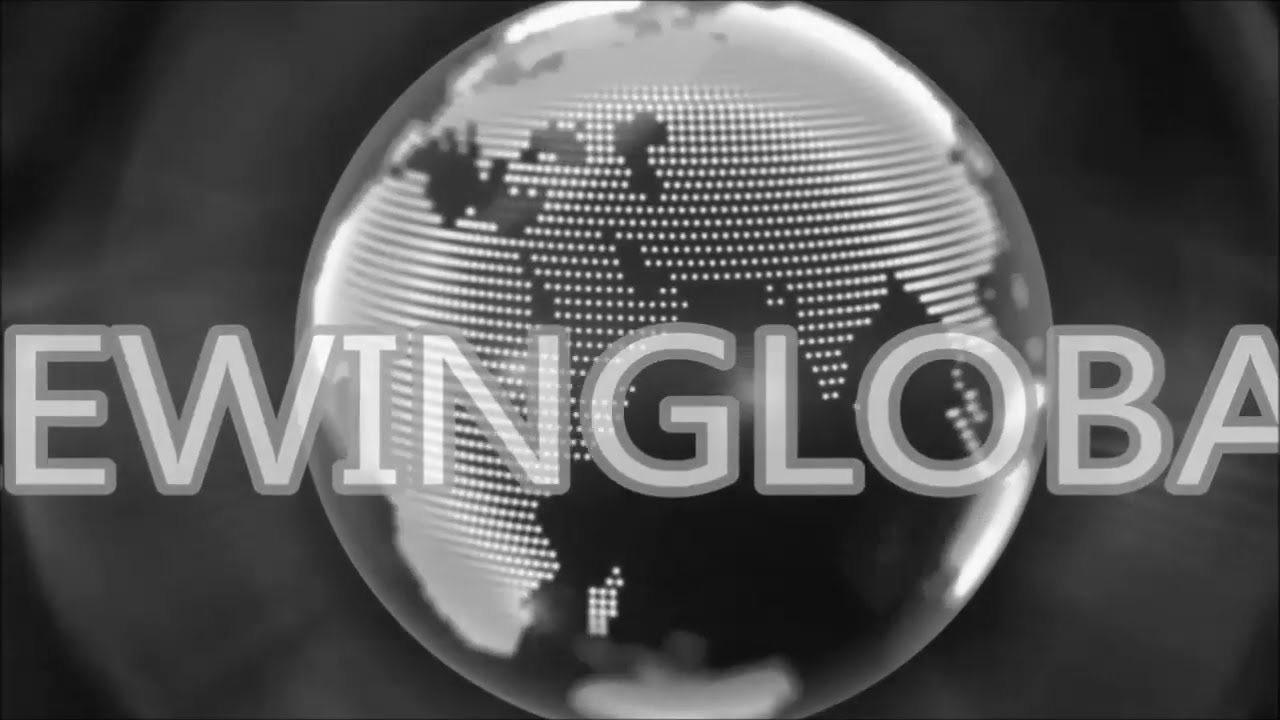This black and white grayscale image features a computer-rendered globe positioned centrally on the page. The globe itself is dark, with the continents represented by rows of white dots, forming a distinct, dotted outline of the land masses. The surrounding ocean areas are darker in contrast. Overlaying the globe is a line of large, capitalized white text that reads "EWINGLOBA," which appears fragmented and might be part of a larger phrase or logo, possibly relating to a media company. The text is bordered by a darker gray outline, adding emphasis. The background surrounding the globe and text is a blurry grayscale, gradually darkening towards the corners, adding depth and focus to the central elements.